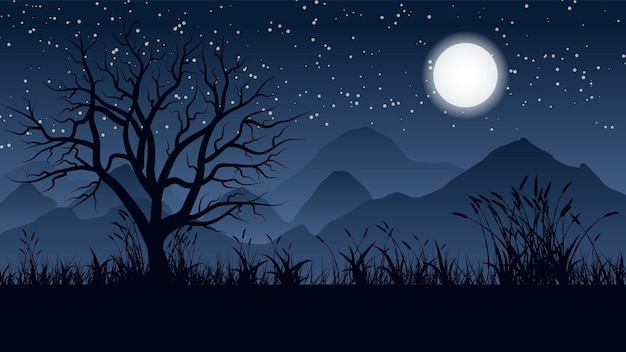A stunning painting captures the serene beauty of a winter night. The composition features a leafless deciduous tree prominently in the foreground, its dark silhouette contrasting against a gradually fading blue sky. The sky is a canvas of star-filled wonder, with countless white dots scattered across the top. A bright, full moon resides in the upper right-hand corner, encircled by a delicate halo, casting a ethereal glow over the scene. Below, cattails grow, adding an element of life to the otherwise stark winter landscape. In the distance, a range of mountains stretches across the horizon, creating a majestic backdrop. The combination of the tree, the starry sky, and the moon creates a tranquil and mesmerizing portrayal of a winter night.